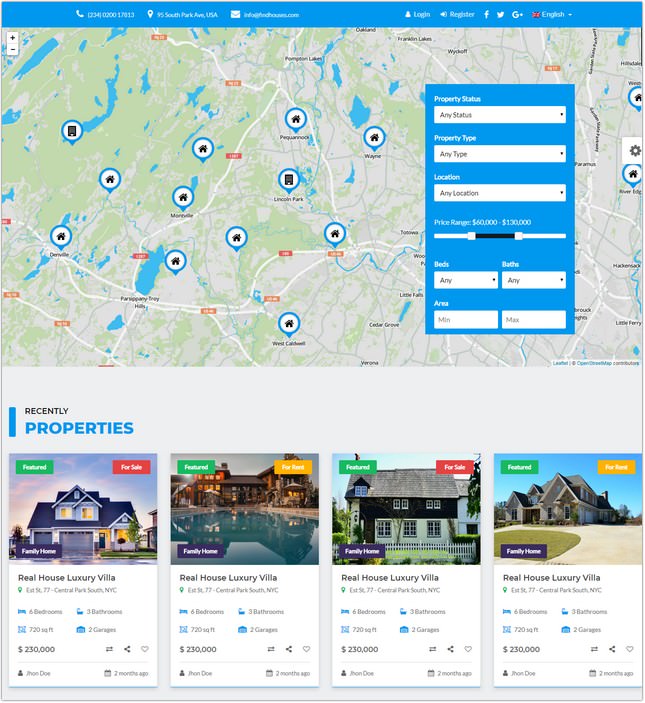The image showcases a webpage dedicated to browsing resort or accommodation options. At the top, there is a section displaying a telephone number and location details, albeit in a small font. 

On the right-hand side, there are additional elements, although they are not detailed in the description. At the bottom of the webpage, an interactive map is shown, highlighting multiple locations with various icons.

Below the map, a section labeled "Recently Viewed Properties" is visible. This section features several listings, mostly labeled as "Real House Luxury Villa." The properties are differentiated by price and features. The first property is priced at $25,000 and resembles a typical family home. The second property, listed at either $250,000 or $230,000, is a villa with a swimming pool. The third listing is a smaller home, while the fourth showcases a larger residence. Each property varies in size and amenities, catering to different preferences and budgets.